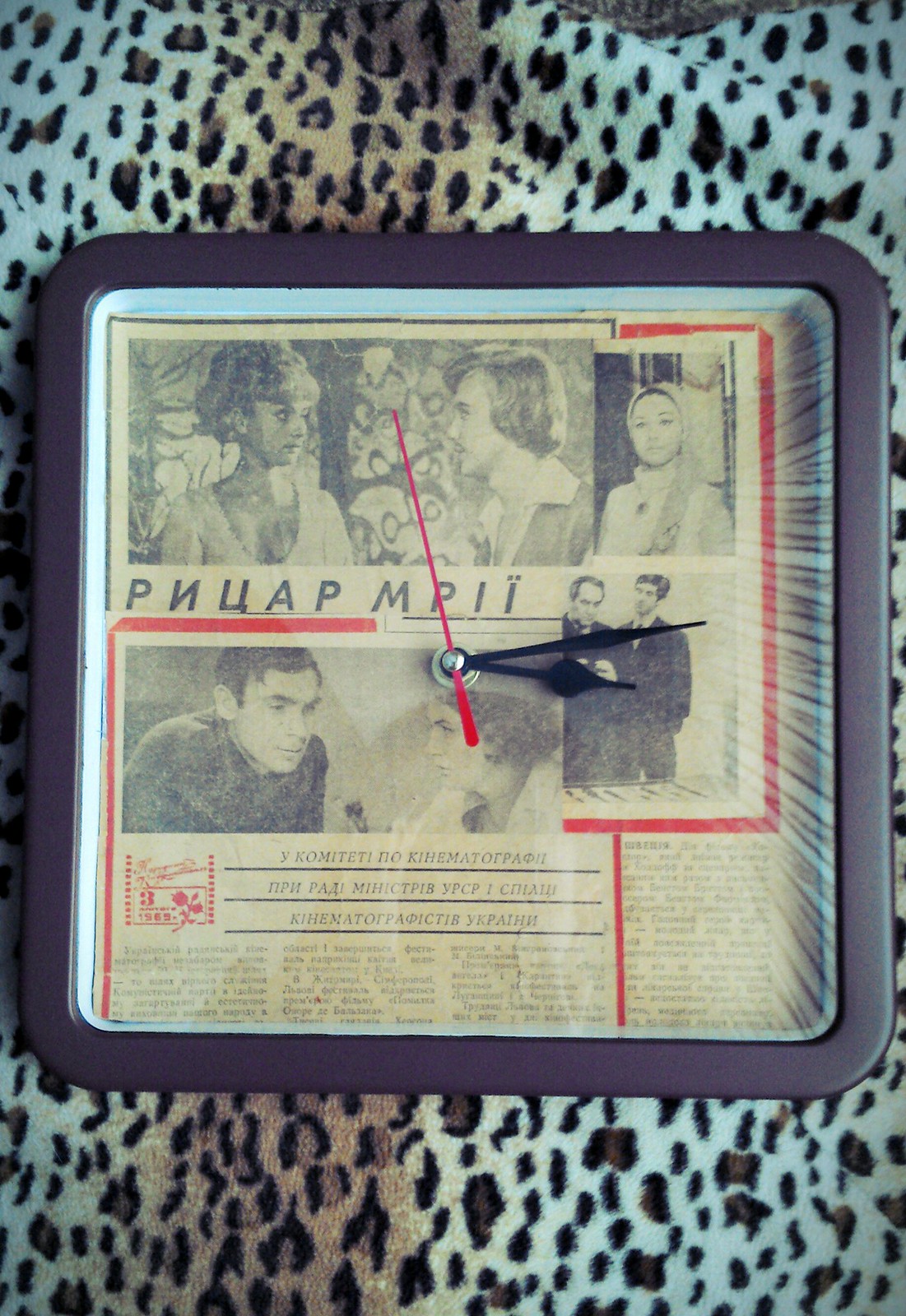The image shows a square clock with rounded edges, framed in dark brown wood, set against a leopard print background in shades of off-white, black, and brown. The clock face resembles an old-fashioned newspaper print with no numbers, and it features black hour and minute hands along with a red second hand. The clock's design prominently includes an off-white poster with red framing and black-and-white images, as well as text written in Cyrillic. The poster appears to state "Roots are mri," and displays two landscape-oriented images stacked vertically. The top image depicts a man and a woman looking at each other, while the bottom image shows two men. Below these images are sections of black text resembling newspaper articles, intersected by vertical red lines.